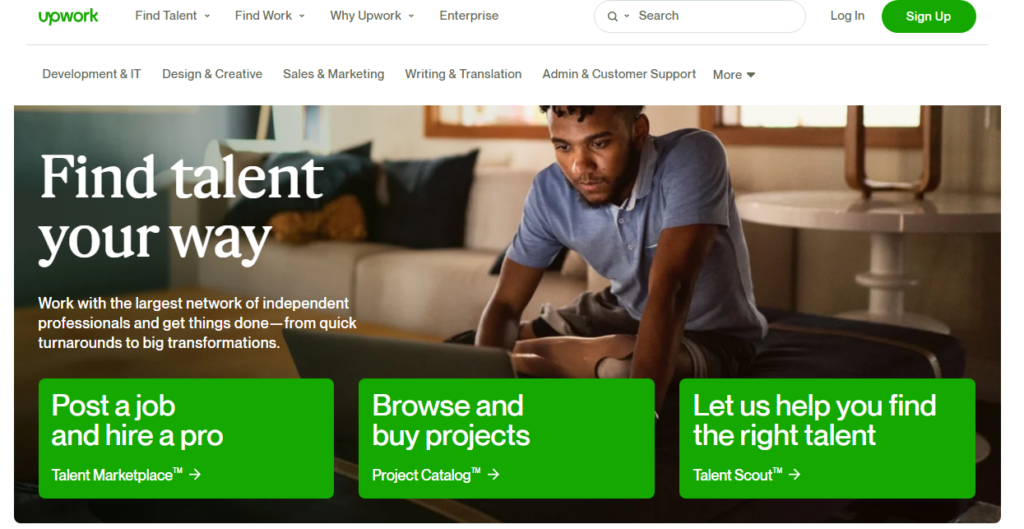The image showcases a webpage from the Upwork website. Against a white background, the upper left-hand corner features the Upwork logo in green. Adjacent to the logo, various navigation tabs are displayed in black, including "Find Talent," "Find Work," "Why Upwork," "Enterprise," and "Talent Scout." The search box is outlined in gray with a white interior, containing a gray magnifying glass icon and the word "Search" next to it. To the right of the search box, the option to "Log In" is presented in black, followed by a green oval button with the text "Sign Up" in white.

A thin green line separates the header from the rest of the page content. Below this line, additional navigation tabs appear in black: "Development and IT," "Design and Creative," "Sales and Marketing," "Writing and Translation," "Admin and Customer Support," and more.

The main section of the page features an image of a brown-skinned man wearing a pale and periwinkle short-sleeved shirt, intently working on a laptop. To the left of this image, bold white text reads, "Find Talent Your Way." Below this, a tagline is visible: "Work with the largest number of independent professionals and get things done. From Quick Turnarounds to Big Transformations."

At the bottom of the page, three green rectangles contain white text: the first rectangle states "Post a Job and Hire a Pro Talent Marketplace," the second one says "Browse and Buy Projects" with a subheading "Project Catalog" and a white arrow pointing to the right, and the last rectangle reads "Let Us Help You Find the Right Talent" with a subheading "Talent Scout" and another white arrow pointing to the right.